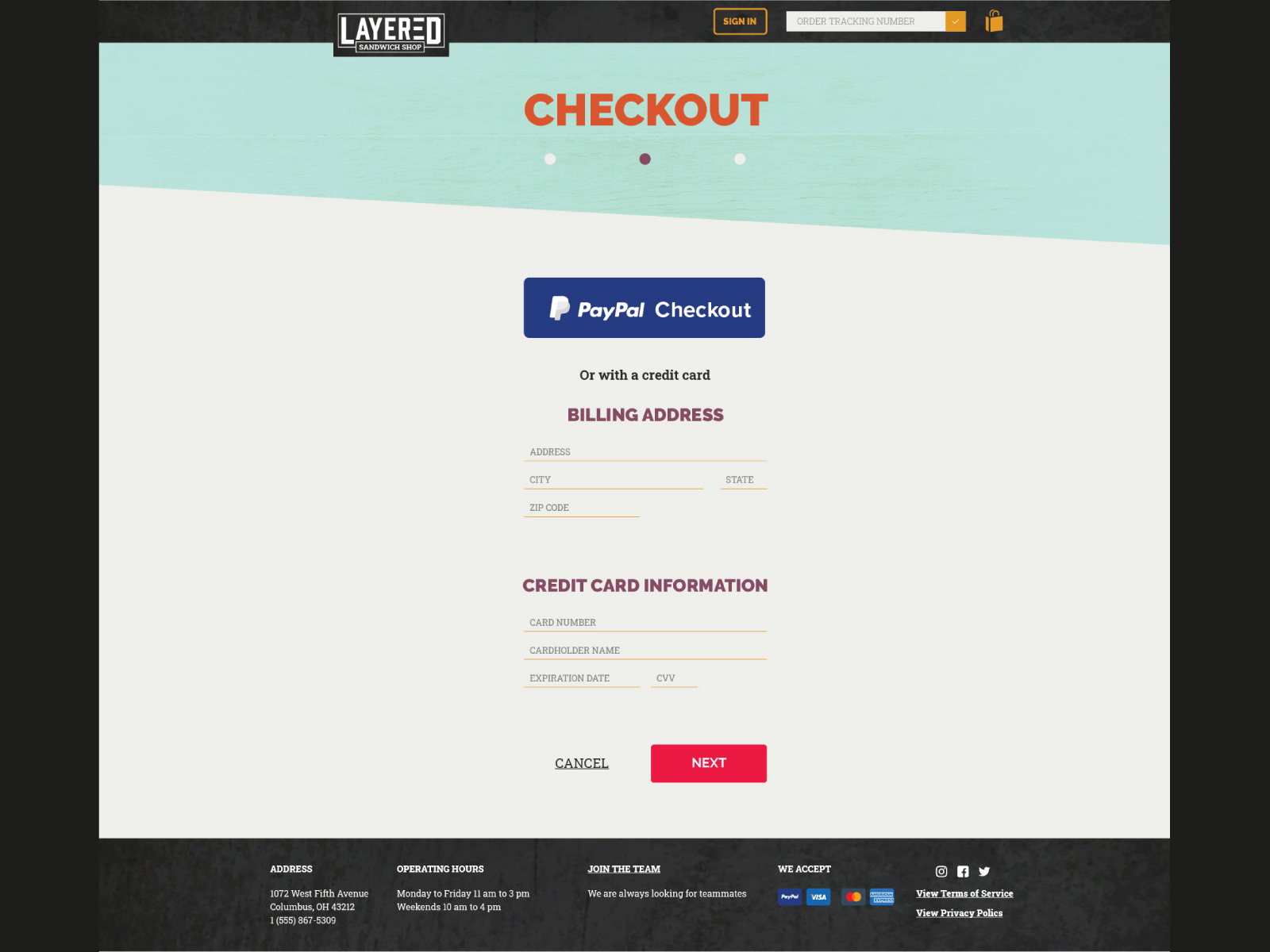The website features a sophisticated design characterized by distinct borders: a medium black border at the top and thicker black borders around the sides and bottom. At the top of the webpage, there is a search bar alongside a sign-in option. Positioned above these elements is a small black rectangle outlined in white trim, displaying the term "layered D" in the center.

The main content area of the site is dominated by a large rectangle, taking up most of the screen. This section has a primarily white background. At the top of this rectangle, there is a banner that widens from left to right and is colored in a light mint shade. Centrally located on this banner, the word "CHECKOUT" is prominently displayed in red, capitalized letters.

In the upper section, there are three clickable dots, presumably indicating different stages of the checkout process. Below this, the options for payment methods are presented: a blue rectangle for PayPal checkout and an alternative for credit card payment. The request for billing address details is highlighted in dark red, followed by fields to input this information, as well as fields for credit card details.

Towards the bottom of this section are two buttons: a "Cancel" button and a red "Next" button for proceeding to the next step. Additional information is available at the bottom within the thick black border.